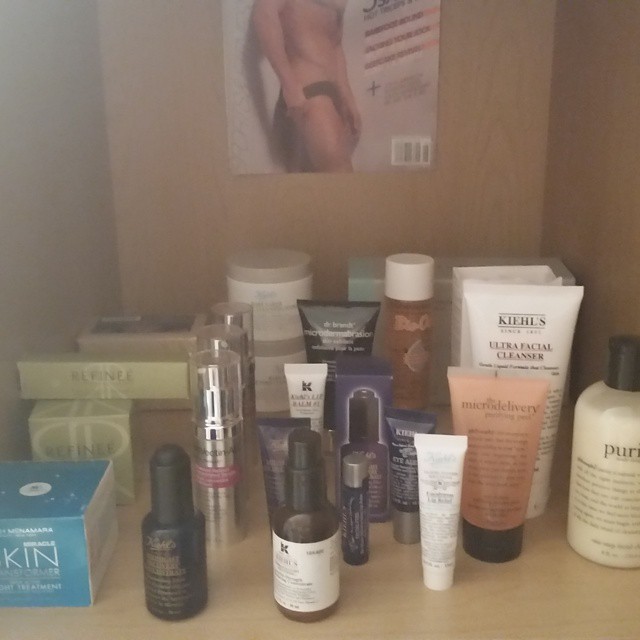The image depicts the interior of a dimly-lit wooden cabinet, stocked with an assortment of skincare and cosmetic products. While the photograph is not particularly sharp, one can make out the presence of a slightly provocative poster placed on the top shelf, featuring a man seemingly removing a thong. Though the text on the poster is unreadable, it adds a risqué element to the scene.

The main focus of the image is the collection of skincare products organized in three to four rows, totaling around 15 to 20 items. Among the array are unopened bars of soap, mascara tubes, small eyedropper bottles of oil, and aerosol spray cans. The collection includes a variety of products such as cleansers, lotions, and skin oils, with packaging colors ranging from white to purple, silver, and black. The packaging design appears gender-neutral, indicating the items are suitable for all genders.

Overall, the image provides a glimpse into a personal skincare collection housed in a wooden cabinet, juxtaposed with a cheeky poster, creating an intriguingly eclectic visual.